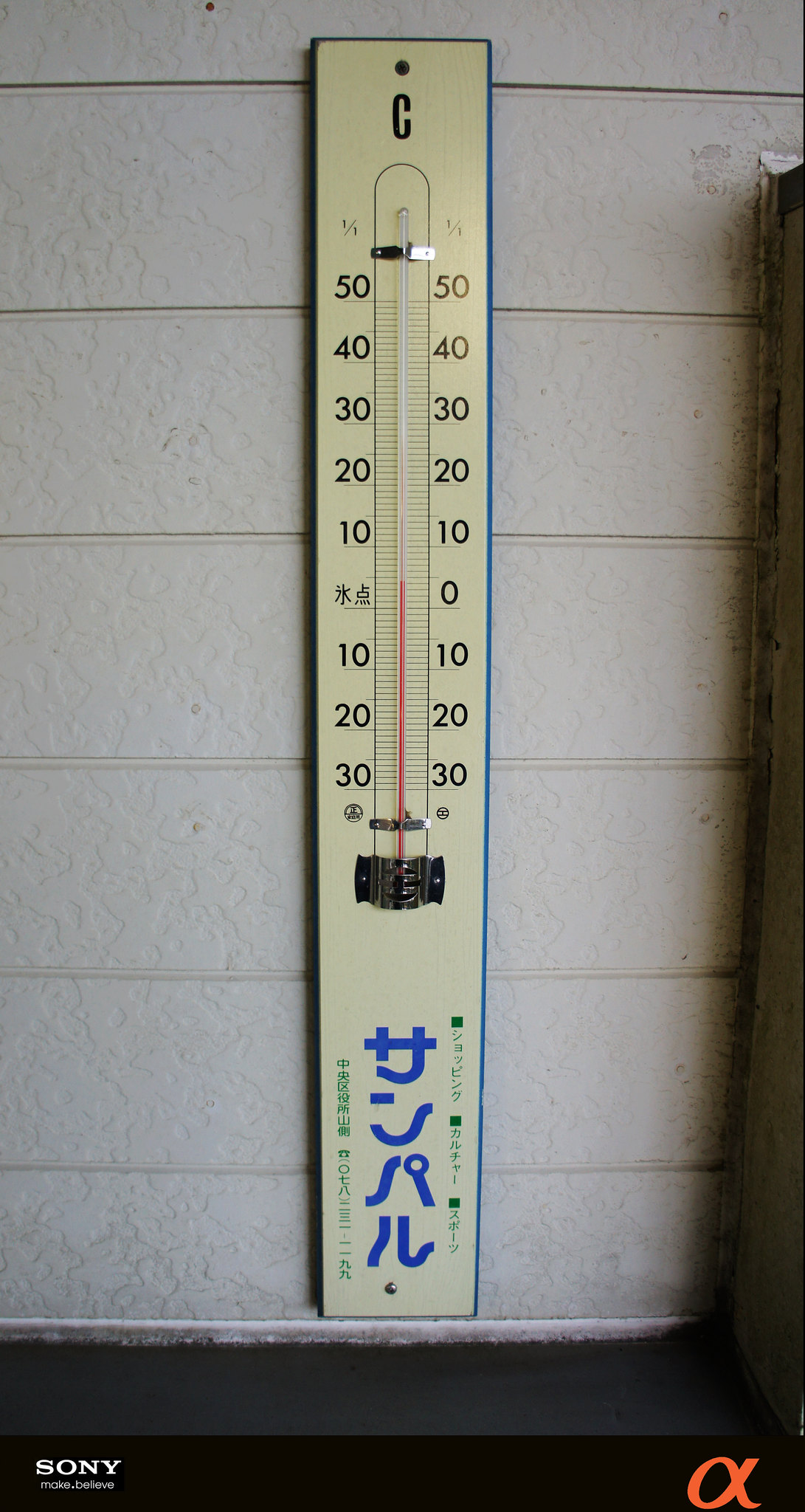The image depicts a wall-mounted thermometer against a white surface, possibly the side of a house. The thermometer displays temperatures with identical numerical scales on both the left and right sides, ranging from at least zero to five degrees with a red indicator currently pointing at five degrees. Unique to this thermometer, the zero mark on the right side is written as a numeric "0," whereas, on the left side, the zero is denoted by two East Asian characters, potentially Chinese or Japanese for "zero."

Below the temperature scale, there are several segments of text. At the center, a large blue inscription is visible, accompanied by smaller green text flanking it on either side. The bottom left of the thermometer features the Sony logo, while the bottom right displays an orange Alpha logo. The thermometer is mounted on a separate black base which secures it to the wall.